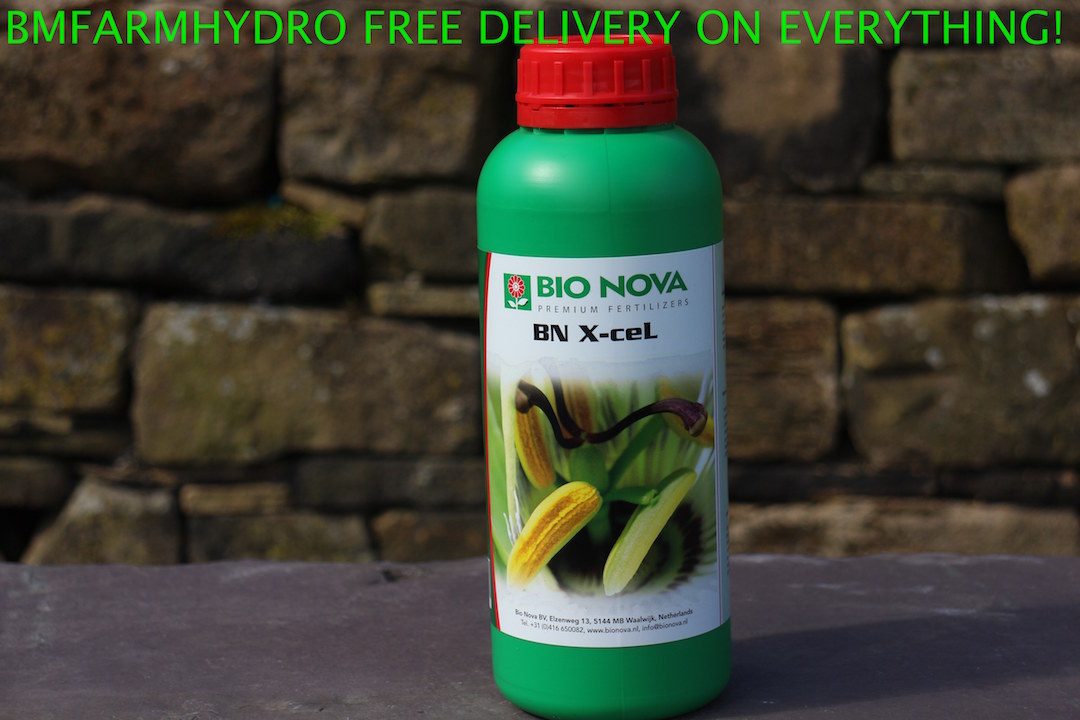In this image, a bottle of Bionova Premium Fertilizers sits prominently on a blackish stone table. The bottle itself is primarily green with a red cap. The label on the bottle features the brand name "Bionova" in large green text, accompanied by an image of a red flower inside a green square. Below the brand name, additional text reads "BNXL," beside which are illustrations of yellow buds that haven't fully bloomed. At the top of the label, there's an inscription "BM Farm Hydro, Free Delivery on Everything!" printed in green, uppercase lettering. The background showcases a textured wall comprised of various shades of tan and brown stones, occasionally marked by blackish and whitish spots, giving it a rustic appearance. The stone table casts a shadow and the bottle reflects some light, indicating that it is a sunny day.